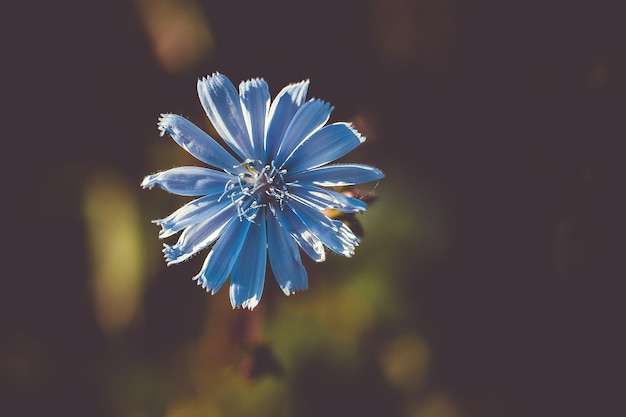The image is a close-up photograph of a delicate flower with intricately detailed, thin petals. The flower exhibits an unusual but captivating periwinkle or light blue hue. Each petal appears slightly frayed or tattered at the edges, resembling a daisy with roughly 20 petals. The zoomed-in focus accentuates the flower's subtle beauty, while its center displays a cluster of small periwinkle and very light yellow or white stamens branching out. The background is a blurred mix of dark green and brown tones, emphasizing the flower's intricate structure and unique coloration in the foreground. The lighting highlights parts of the flower, adding depth and a slightly shaded effect, enriching the overall visual appeal.